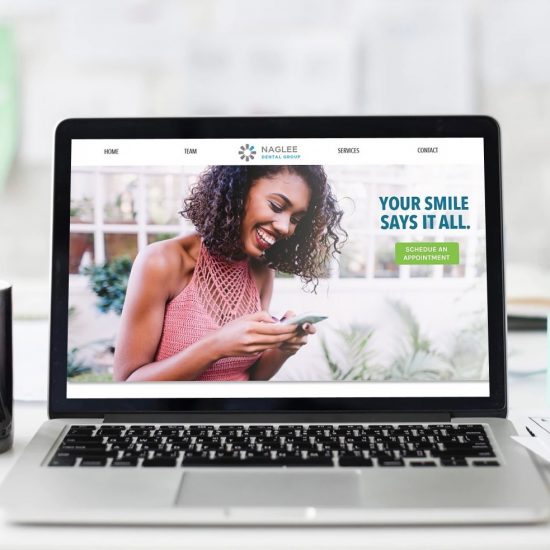A silver-colored laptop or Chromebook is featured in this image, with its sleek metallic finish providing a modern aesthetic. The keyboard, comprised of black, square, and rectangular keys, stands out against the silver backdrop. On the screen is a vibrant picture of a young woman, potentially of African American descent, with curly black hair and toned arms. She has a warm, brownish-tan complexion and is captured in a candid moment, smiling broadly, almost laughing, as she looks at something on her phone. She is dressed in a knit tank top with woven detailing at the top. The setting suggests she is seated, surrounded by plant life and windows that allow natural light to filter in.

At the top of the screen, the website’s navigation bar is visible, with options like "Home" and "Team" on the left. In the center, "Nagli Dental Group" is prominently displayed in text, accompanied by a floral icon. Additional options, including "Services" and "Contact," are positioned to the right. Beneath the navigation bar, a catchy tagline reads, "Your smile says it all," followed by a call to action: "Schedule an appointment."